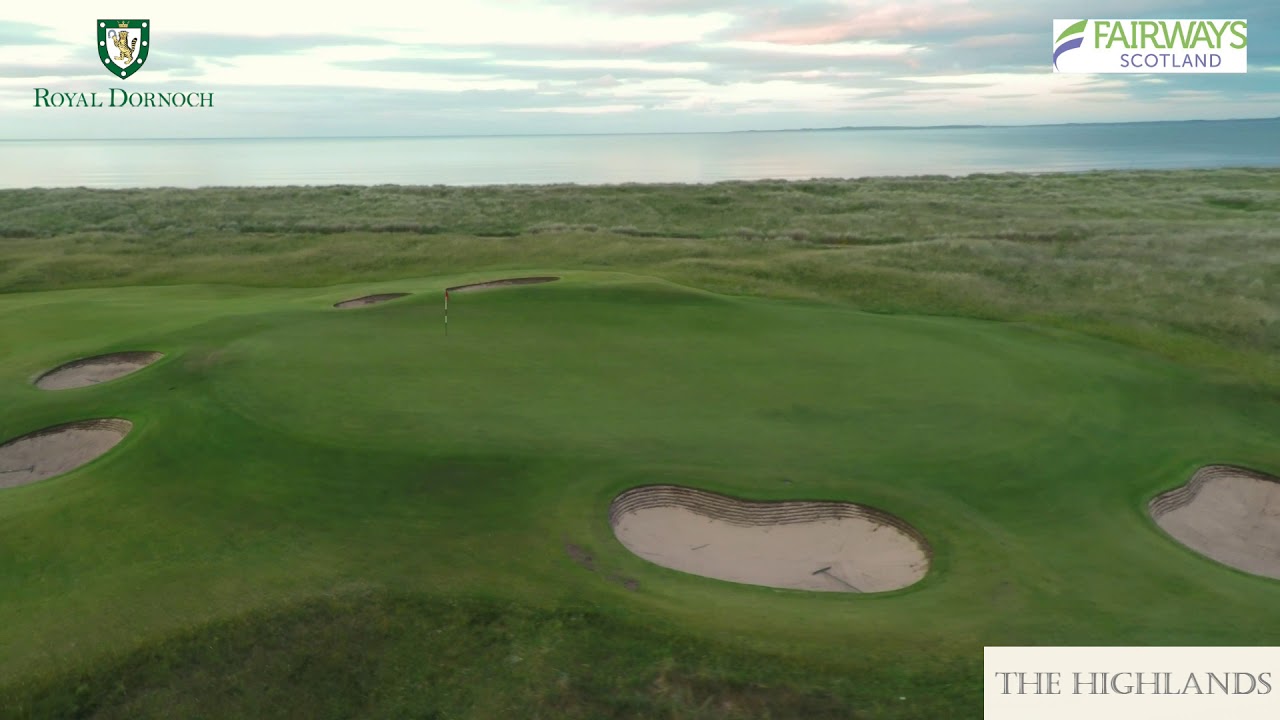The image captures a scenic advertisement of a golf course situated in the Highlands of Fairway, Scotland. The upper left corner features a green and white shield-shaped watermark with an emblem resembling an animal wielding a golf club, branded with the text "Royal Dornoch" beneath it. In the top right corner, another insignia displays "Fairways" in green and "Scotland" in blue. The bottom right corner contains the text "The Highlands" in black on a white background. The sky above is cloaked in a mix of white and blue clouds, evoking the impression of water along the horizon. The foreground reveals a meticulously maintained green field with several tan-colored sand pits and a flag marking a hole, emphasizing the classic features of a traditional golf course.